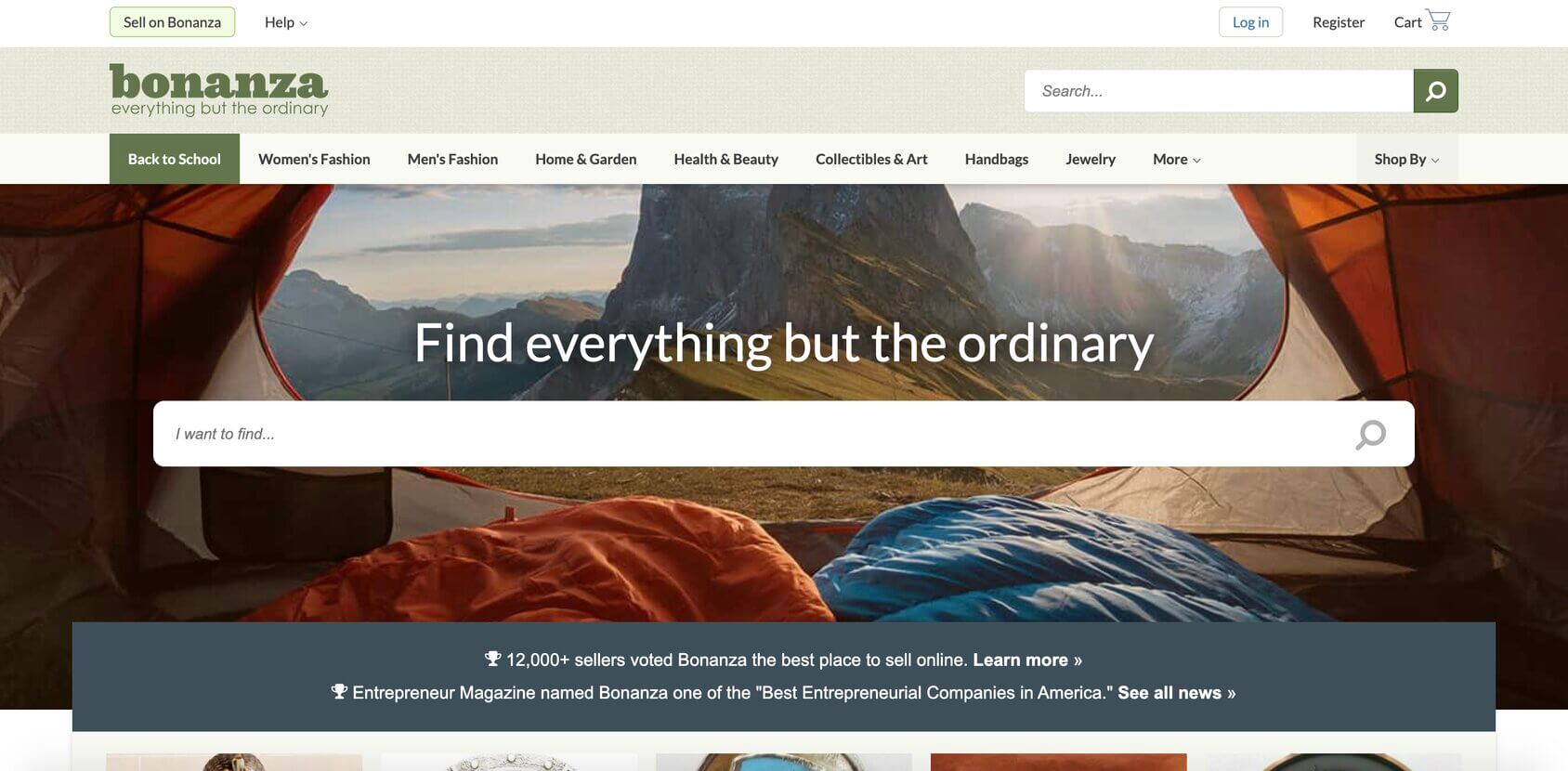This is a screenshot from the website Bonanza, a platform for buying and selling items. The page features a header with a minimalistic white menu, including options for Help, Login, Register, and a Shopping Cart icon on the right side. The Bonanza logo, displayed in green text on a gray background, is prominently positioned. To the right is a wide search bar accompanied by a green search button.

Below the header, there's a primary navigation menu. The first tab, "Back to School," is highlighted with a green background, while other options like Women's Fashion, Men's Fashion, Home & Garden, Health & Beauty, Collectibles & Art, Handbags, Jewelry, and others are on a white background. This menu allows users to shop by various categories via a dropdown.

The central image in the screenshot captures a view from inside an orange tent, showcasing both orange and blue sleeping bags. The tent is partially open, revealing stunning mountainous scenery bathed in sunlight. The caption within the image reads "Find everything but the ordinary," positioned above a wide search bar that spans almost the entire width of the site. Text within the search bar states, "I want to find..."

At the bottom of the screenshot, promotional text highlights Bonanza's selling features: "12,000 sellers" and "Bonanza: the best place to sell online. Learn more." It also mentions that Entrepreneur magazine named Bonanza one of the best entrepreneurial companies in America, encouraging users to "See all the news." The lower part of the screenshot hints at image thumbnails, but they are cut off and not fully visible.